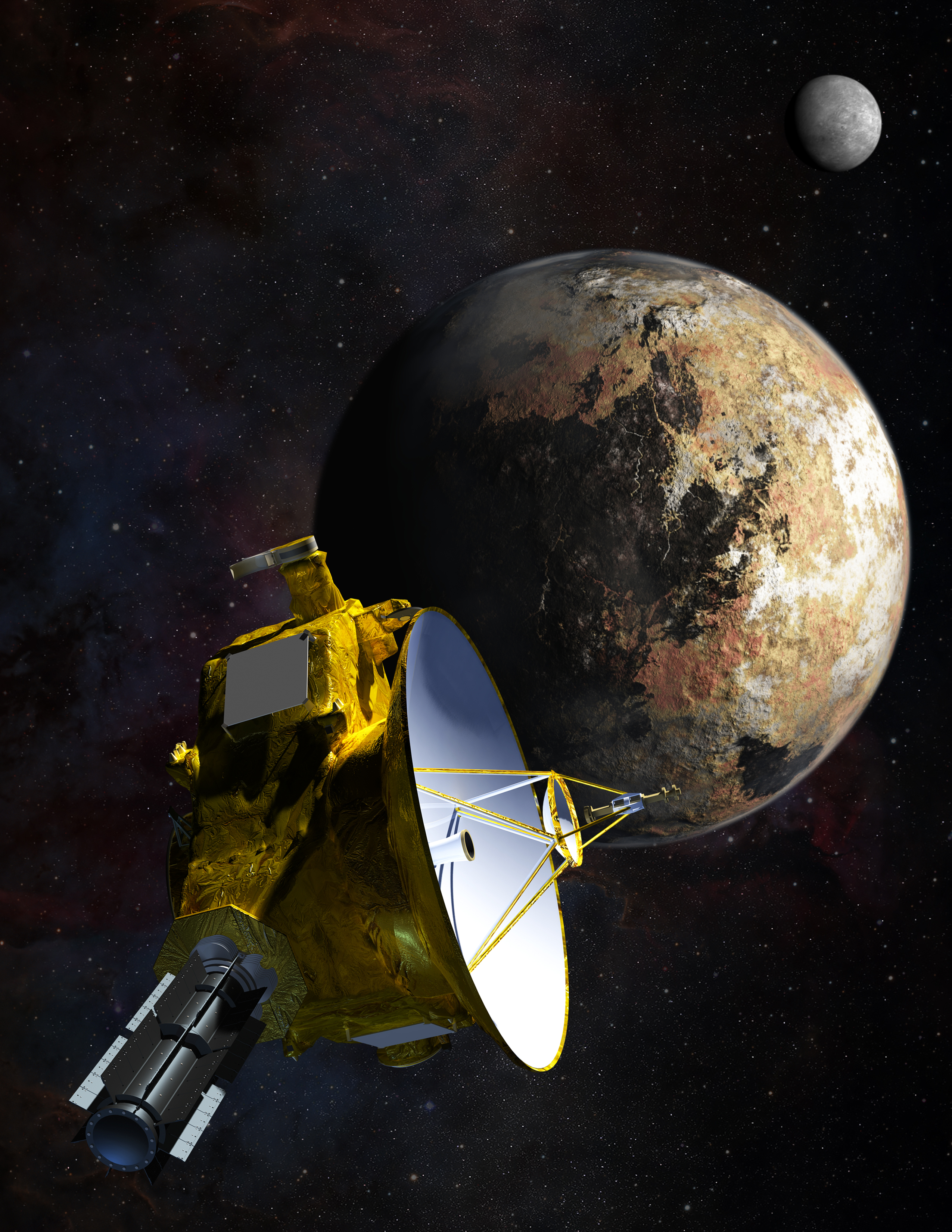In this captivating image of outer space, the vast expanse of the galaxy serves as a backdrop, predominantly black with scattered white dots resembling distant stars. Hints of red add a touch of color to the scene. In the upper right corner, a small, circular, solid grayish sphere can be observed, likely representing a distant moon. 

Centrally, there is a planet, though its identity is ambiguous due to its unusual color palette of black, gray, orange, and red, possibly suggesting an artistic rendition of Earth rather than a realistic depiction. 

Foregrounded prominently is a large satellite. The satellite's exterior is a vibrant yellow, while its core is primarily white. Extending from this central white section are yellow poles, adding intricate detail to the structure. The satellite's design and coloration contrast starkly with the cosmic background, making it a striking focal point in the image.